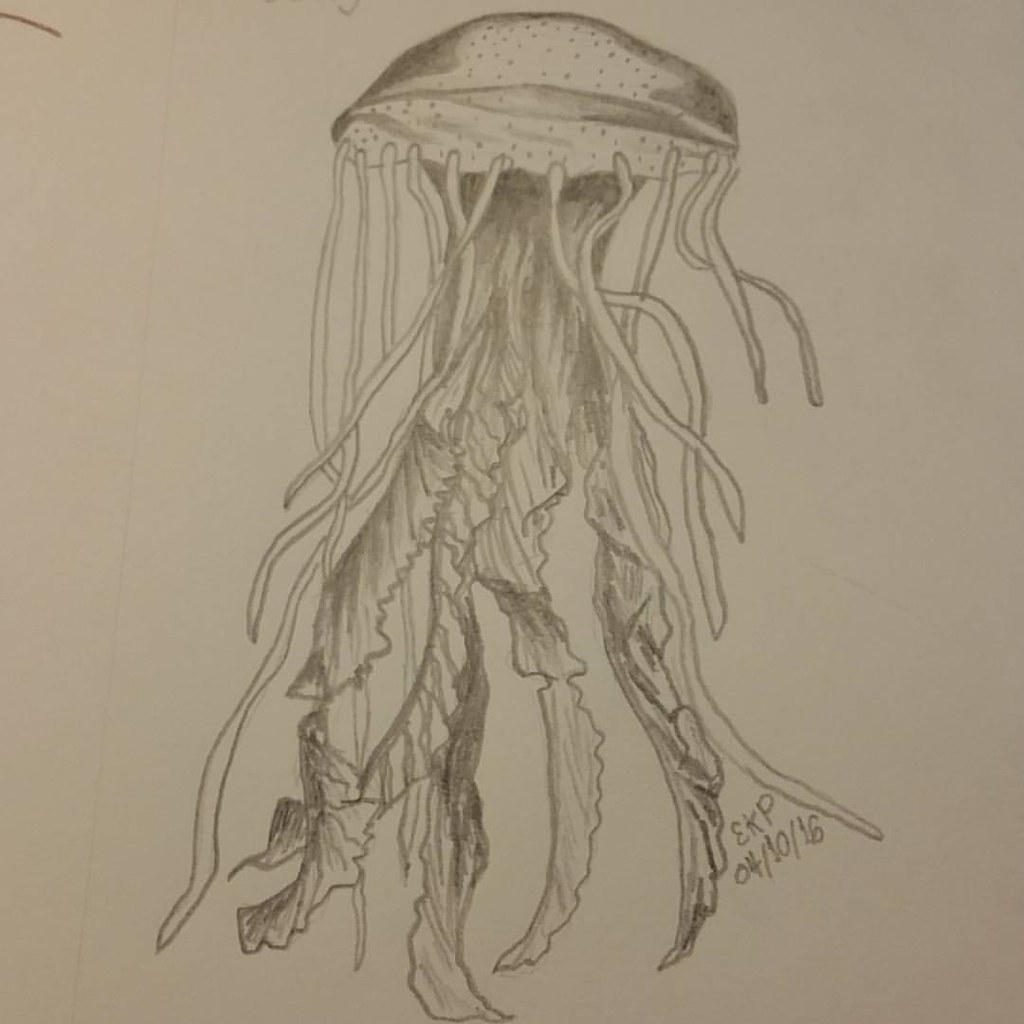This is a highly detailed pencil drawing of a jellyfish, executed on off-white, square sketch pad paper. The jellyfish's body starts at the top center of the page, forming a half-moon or rounded shape, fully adorned with polka dots. The edges of the body are darkened for emphasis. Emerging from the body are numerous tentacles, appearing like long, narrow snakes, suggesting movement as if they were undulating in water. At least ten delicate tentacles extend from each side of the body. In the middle section, there are darker-shaded, thicker pieces that resemble seaweed or strings of lettuce, adding depth and texture to the creature's appearance. In the bottom right corner of the page, beneath a tentacle, is the text "EKP" followed by the date "04/10/16," indicating the work was created on April 10, 2016. Overall, the artistry captures the ethereal yet potentially dangerous essence of a jellyfish.